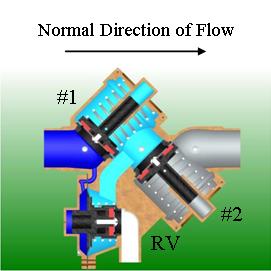The image features a detailed diagram against a green background, illustrating a complex piping system. At the top, bold black text reads "Normal Direction of Flow" with an arrow indicating the flow direction from left to right. The central focus is a set of three interconnected pipes entering from different directions: the left, the bottom, and the right. Each pipe connects to a central pump-like diagram that contains a red cylindrical component blocking the respective pipe.

The pipe on the left, labeled "1," is dark blue in color. The bottom pipe, which is white, is labeled "RV." The right pipe, labeled "2," is gray. The connection point of these pipes features blue liquid within the intersecting sections between the pump-like diagrams. The overall color scheme includes shades of blue, gray, and white, set against the green background, detailing the path and structure of this intricate piping system.